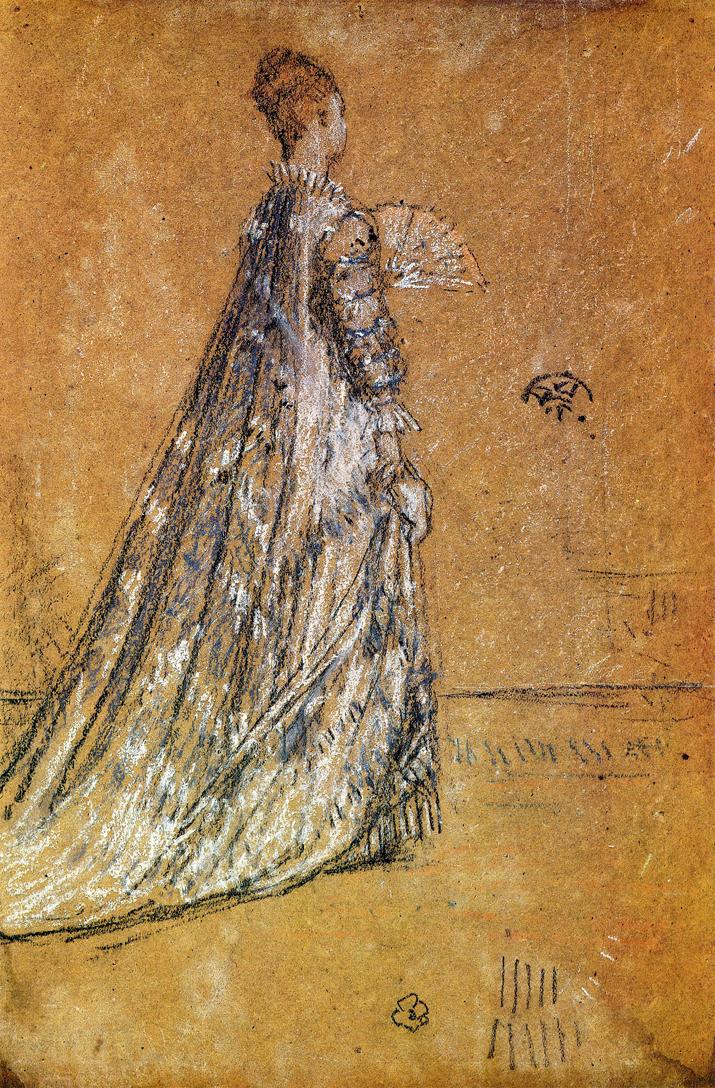This image is a detailed oil painting titled "The Blue Dress" by James McNeill Whistler, created in 1871. The artwork, done in an Impressionist style, features a woman in profile facing towards the top right. Set against a light, gold-brown parchment-like background with random sketch marks, the woman stands out prominently. She is elegantly dressed in a formal gown that cascades to the floor with a long train. The gown is adorned with intricate embroidery in beige, black, and gold tones, accented by white highlights. Her arms are covered with long, puffy sleeves ending in white lace at the wrists. A white lace glove adorns her right hand, which rests at her side. Her left hand gracefully holds an ornate, fanned-out fan with gold and white highlights, evoking an aesthetic reminiscent of the Far East. Her reddish-brown hair is styled into a bun on top of her head, complementing the darker tones contrasting against the golden background. Symbolic elements, including indistinct figures and a possible chair appear towards the front of her in the composition, adding layers of intrigue. The painting is rendered in a style that blends elements of both sketches and finished works, giving it a timeless and historical feel.